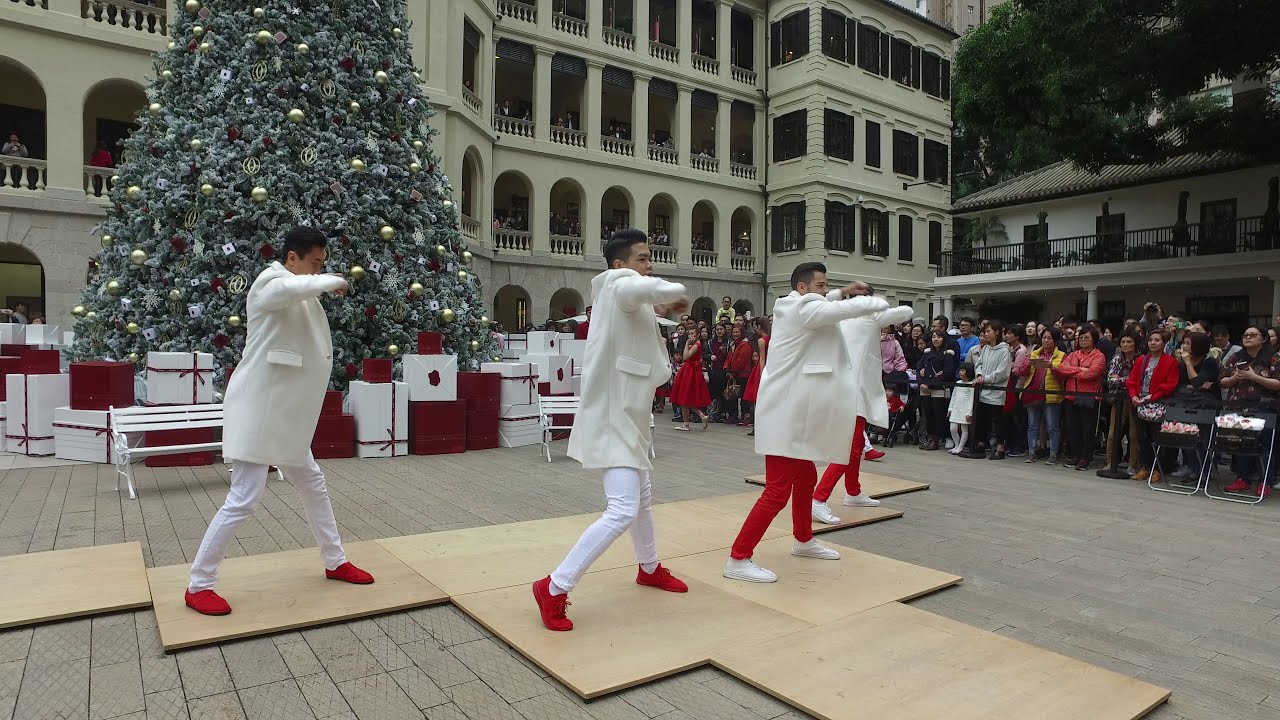In a bustling town square, a lively Christmas performance unfolds in front of a grand, tall building with four visible floors, though the bottom one is obscured by the festive scene. This white-ish tan stone building is adorned with rows of small arches and balconies, complete with elegant rail guards and black squared windows at the far right edge. The building serves as a backdrop to a beautifully decorated, dark green Christmas tree dusted with snow and adorned with golden and silver ornaments. Bags and presents, wrapped in white with red ribbons and burgundy touches, are scattered around the tree, enhancing the holiday spirit.

In front of the tree, four performers dressed in coordinated outfits add to the lively Christmas atmosphere. The dancers, likely young men, are clad in white jackets, with two wearing white pants paired with red shoes and the other two in red pants with white shoes. They execute synchronized dance moves on a specially laid-out floor of wooden tiles, distinct from the brick-paved square. Their dynamic poses, with bent arms, enhance the festive mood.

To the right, a crowd of spectators watches intently from behind a black safety line, absorbing the visual feast. The entire scene is bathed in the warmth and joy of the season, creating a vibrant tableau of holiday celebration.